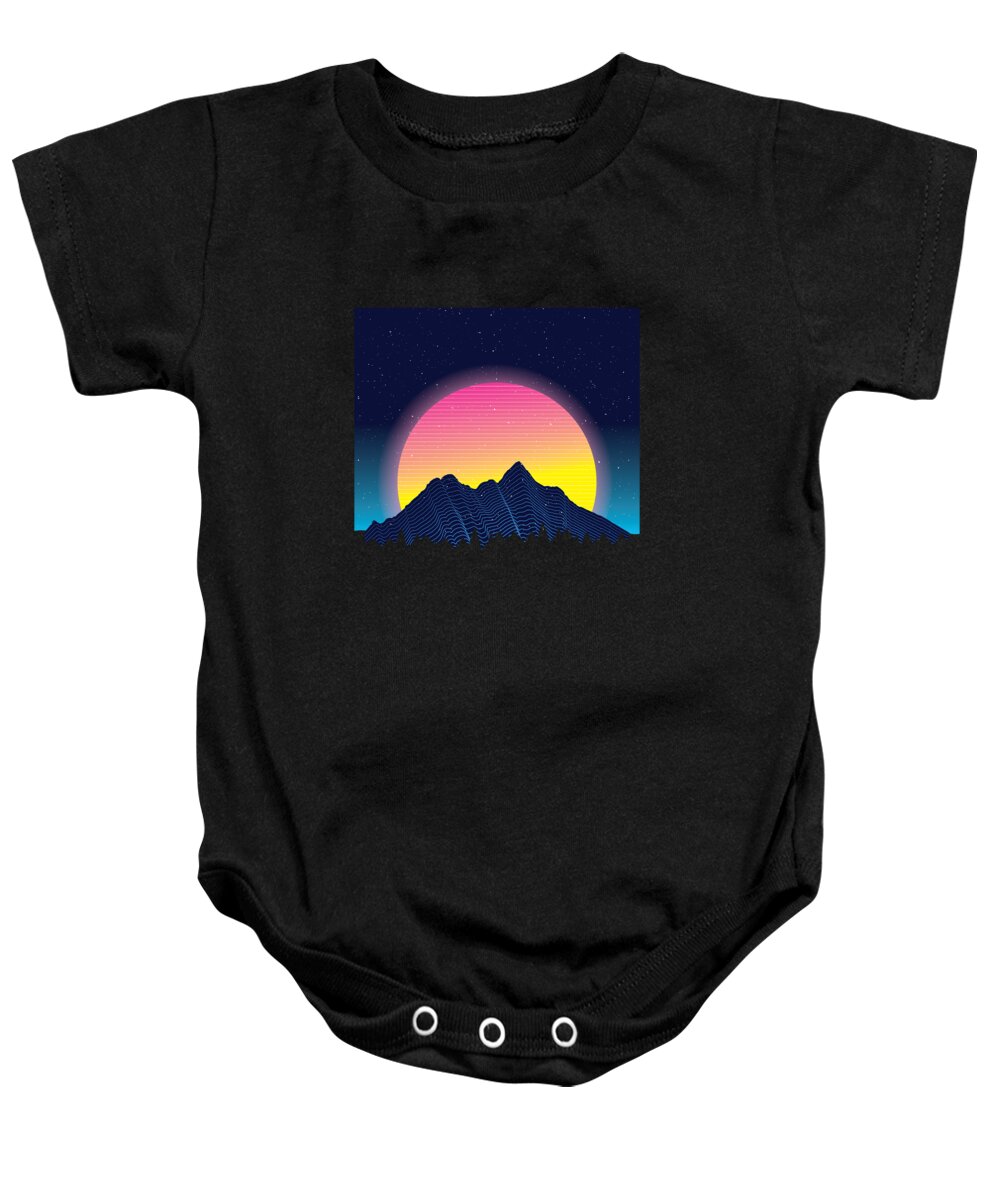The image features a black infant onesie with short sleeves and a ribbed collar, displayed against a plain white background. The onesie has three silver snaps at the bottom between the leg holes. Centrally positioned on the chest area, there is a rectangular transfer design showcasing a vivid sunset or sunrise. The illustration within the rectangle depicts dark navy blue mountains with jagged peaks and pine trees at their base. Rising from behind the mountains is a large, radiant celestial body—either the sun or moon. The lower part of this body is a bright yellow, transitioning to a light pink, and then to a deeper pink at the top. Surrounding this celestial body is a light bluish glow. The sky in the illustration features varying shades: a bright blue on the sides near the bottom, transitioning to a darker navy blue with tiny white dots (resembling stars) at the top, creating a striking contrast that highlights both the mountainous landscape and the celestial event.